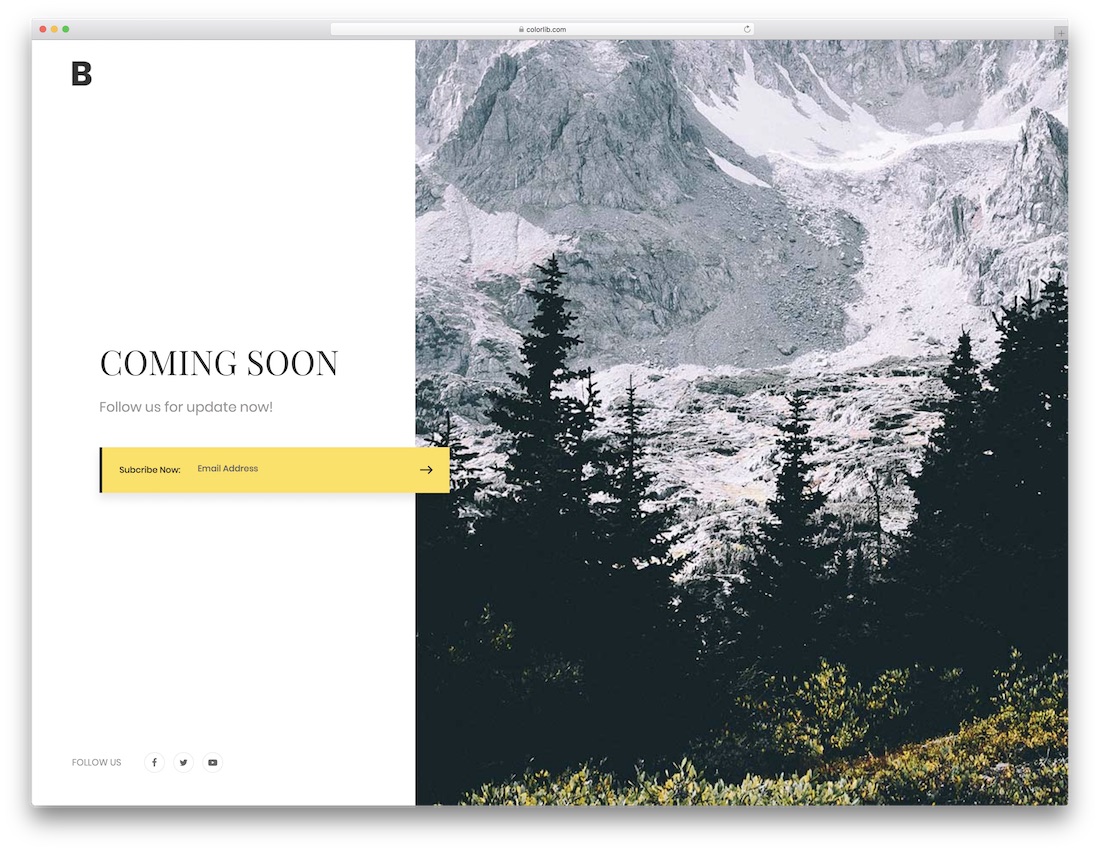A screenshot from an older Mac computer displays a "coming soon" placeholder page on a website. On the left side of the page, a minimalist letter "B" logo is located at the top left corner. Below the logo, centered text reads: "Coming Soon. Follow us for updates," alongside fields prompting visitors to "Subscribe Now" by entering their email address. At the bottom of the page, smaller text encourages users to "Follow Us," accompanied by social media icons for Facebook, Twitter, and what appears to be either YouTube or Instagram.

On the right side of the page, a scenic image depicts the base of a gray-tinted mountain with dark trees lining its base. The trees appear almost black, contrasting with the minimal patch of grass visible at the very bottom of the image. The subdued colors give the scene a somewhat surreal, monochromatic feel, highlighting the mysterious character of this "coming soon" webpage.